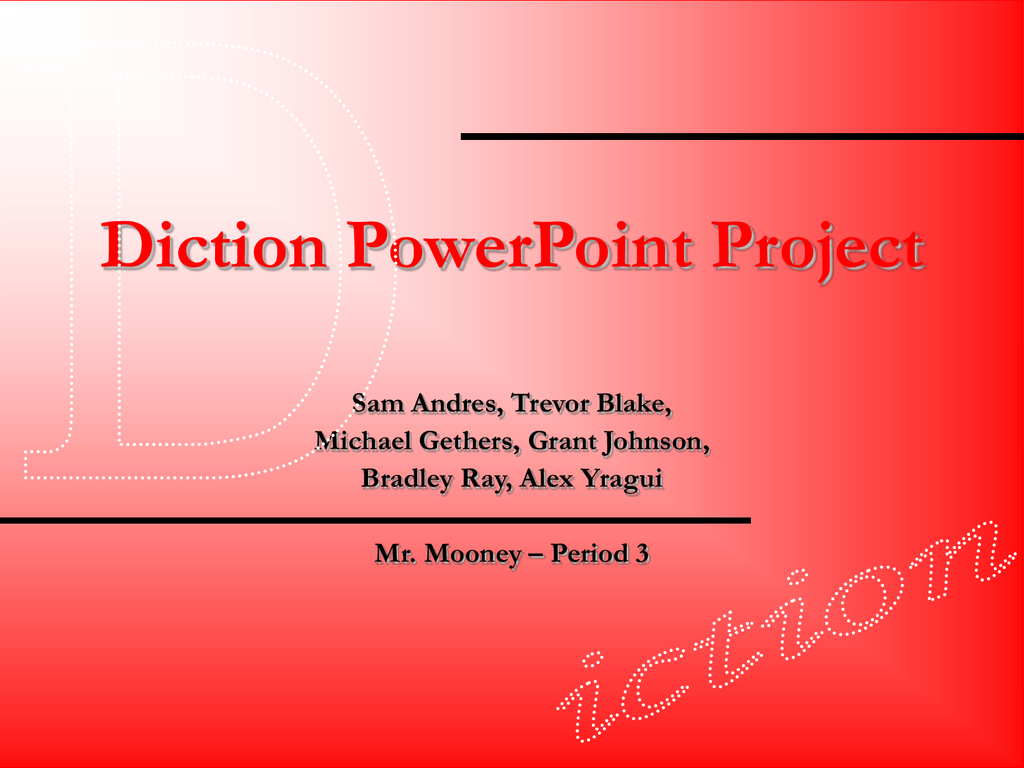The image is a detailed PowerPoint slide characterized by a distinctive gradient background that transitions from white in the top left corner to red in the bottom right. Dominating the upper left of the slide is a large, dotted letter 'D' blending subtly into the backdrop. Centrally positioned at the top, in bold red text, is the title "Diction PowerPoint Project," flanked above and below by horizontal black lines extending partially across the slide. Under the title, centered black text lists the authors: Sam Andres, Trevor Blake, Michael Gethers, Grant Johnson, Bradley Ray, and Alex Iragui, each name stacking line by line. Further below, another black line spans approximately three-quarters of the slide’s width, beneath which sits additional black text, "Mr. Mooney - Period 3." Concluding the visual presentation, the word "Ixion" appears in the bottom right corner, cleverly spelled out in white dotted text at a diagonal angle, completing the 'Diction' theme initiated by the prominent 'D' at the top.